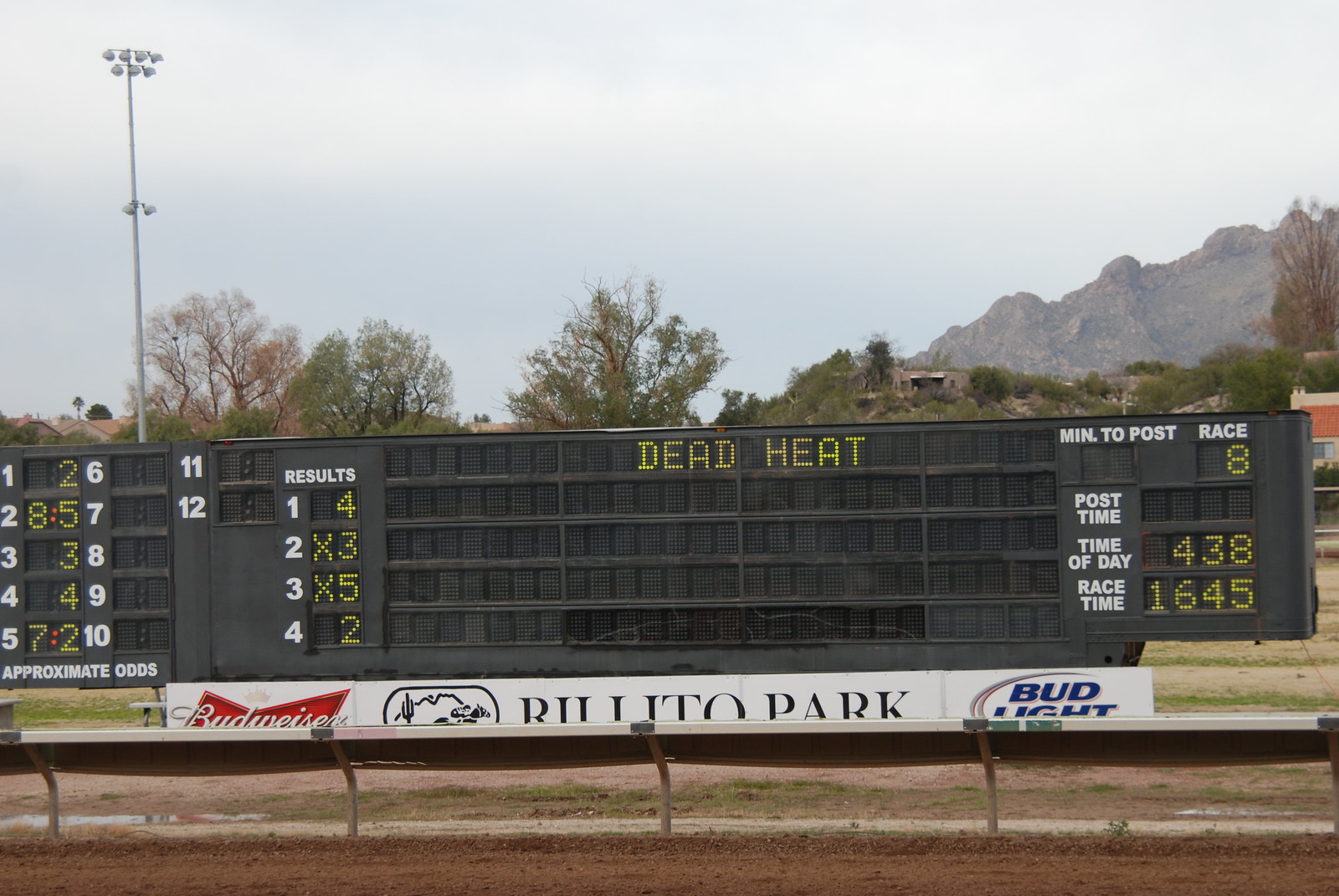The image features a bustling horse racetrack, prominently displaying a large digital scoreboard. The scoreboard, black and rectangular with digital and green lettering, announces a 'Dead Heat' in race 8, with the results showing numbers 4, X3, X5, and 2. The board also lists the approximate odds such as 2, 8 to 5, and 72, along with critical race information including post time at 16:45 and the current time of 4:38. The background captures lush greenery with bushes and trees, juxtaposed against distant mountains and a clear sky. The scene is sprinkled with advertisements for Budweiser and Bud Light. To the left of the sign, a towering white light pole with multiple lights stands tall behind the scoreboard. Surrounding the racetrack is a metal railing enclosing brown dirt, adding to the rustic charm of what appears to be either Rolito Park or Bolito Park, partly obscured by the pole.